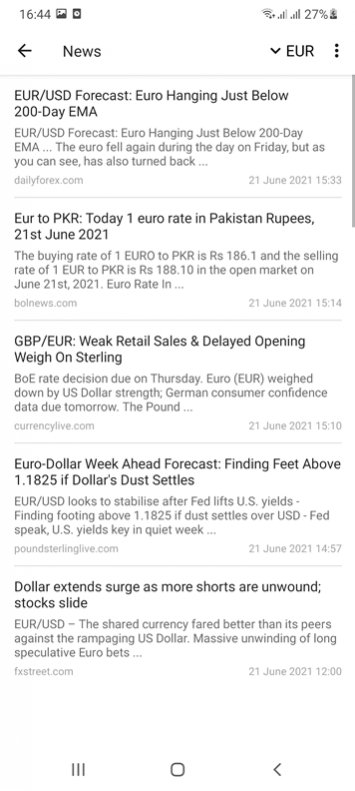This image captures a screenshot of a smartphone displaying a financial news application with updates on currency exchange rates and market activity. At the top of the screen, the phone's taskbar is visible, showing the time, Wi-Fi signal strength, and battery status.

The content of the screenshot begins with a heading labeled "News," followed by a series of articles focused on exchange rate forecasts and related financial insights. The first headline reads, "EUR/USD Forecast: Euro hanging just below 200-day EMA," accompanied by a brief summary stating, "The Euro fell again on Friday but has also turned back." This article is dated June 21, 2021. Another snippet addresses the exchange rate between the Euro and the Pakistani Rupee, indicating, "Today’s 1 Euro rate in Pakistan Rupees, June 21, 2021."

Further down, the news feed provides additional articles, such as, "GBP/EUR: Weak retail sales and delayed opening weigh on Sterling," followed by, "EUR/USD Week Ahead Forecast: Finding feet above 1.1825 if Dollar does settle." The final headline in the visible portion of the screenshot reads, "Dollar extends surge as more shorts are unwound; stocks slide."

The detailed description and dates suggest that the content is focused on providing current and actionable financial information relevant to currency traders and market analysts.